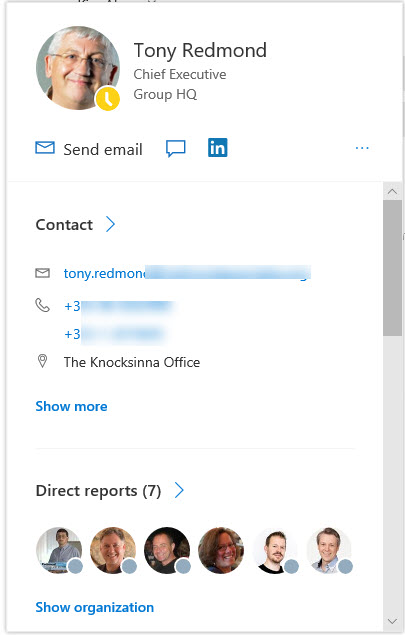In this slightly blurred screenshot, we observe a LinkedIn profile belonging to Tony Redmond, an older white male with gray hair. His circular profile picture is displayed at the top left of the image, showcasing him wearing transparent glasses and a warm smile. A yellow status indicator at the bottom right of the profile picture suggests he is currently busy.

Next to the profile picture, Tony Redmond's name appears prominently in black text, followed by his professional title, "Chief Executive," and his association with "Group HQ." Directly beneath the profile picture, there are icons including an envelope symbol, the text "Send Email," a chat logo, and the LinkedIn logo.

In the middle left section of the image, the text "Contact" is displayed, followed by Tony's contact information. The details include an envelope icon next to his partially redacted email address, a telephone icon with a blurred-out phone number, and a location icon indicating "NAC Sena Office."

At the bottom of the image, there is a section titled "Direct Reports," featuring several additional profile pictures, highlighting other members of the organization connected to Tony Redmond.